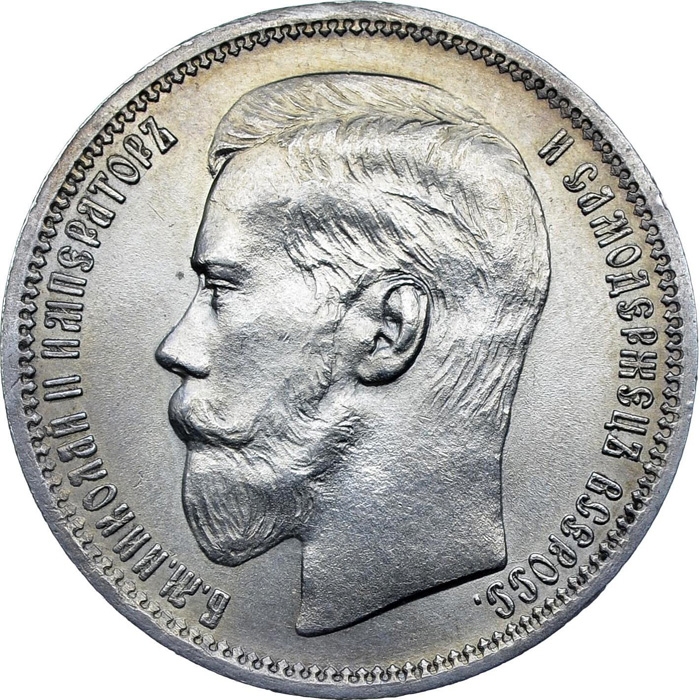This close-up image captures an aged silver coin, which is beginning to show signs of tarnish and rust, particularly along its edges. The coin features a detailed, three-dimensional profile of a man facing left, centrally positioned yet slightly off at the bottom. The man has a neatly trimmed haircut, a long beard extending from his hair down midway through his neck, and a prominent mustache. His expression is stoic and unsmiling, lending him an unfriendly appearance. The coin's exterior is adorned with a saw-tooth engraving all around its circumference. Additionally, there is intricate lettering or numbering along the inner edge of the coin, possibly in Russian or German, although it is difficult to decipher due to its orientation and wear.